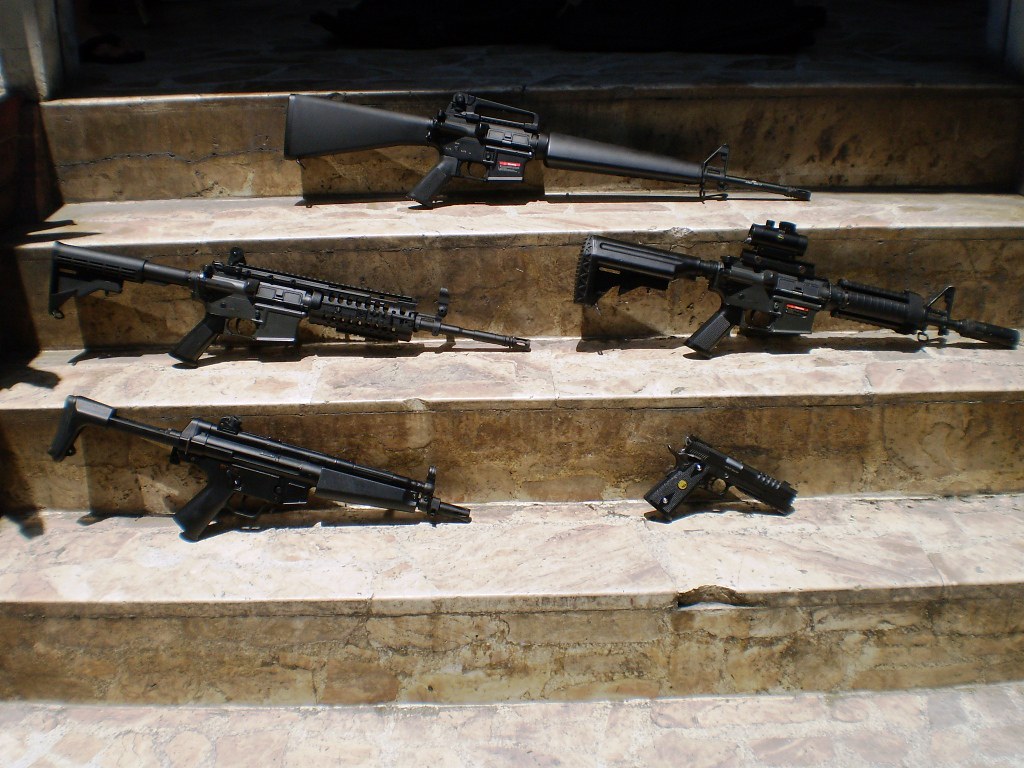The image depicts five black, modern firearms meticulously arranged on a set of sandy, mottled, brown marble steps, leading into a dark, indiscernible doorway. The steps are brightly illuminated with naturalistic lighting, creating distinct shadows beneath each gun. On the lowest visible step, to the left lies a black submachine gun, while to the right sits a black handgun with a short barrel. The next step up features two assault rifles; the one on the right is equipped with a scope. On the third step from the bottom, an especially long-barreled black rifle, possibly a hunting rifle, occupies the center position. All the guns appear new and in pristine condition, contrasting sharply with the aged appearance of the stone steps they rest upon.